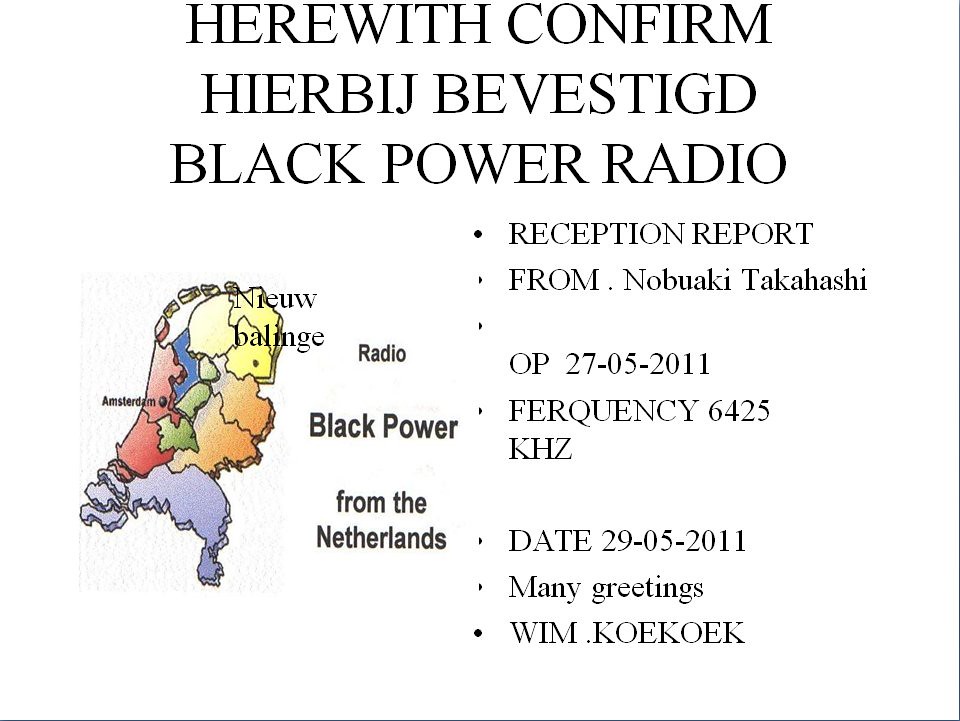The image features a central text on a white background that reads, "Herewith Confirm Herbitch Bephistic Black Power Radio." Below this, it states "Reception Report from Nobuaki Takahashi," alongside the date "29-05-2011" and the frequency "6425 KHZ." The message is concluded with "Many greetings, WIM.KOEK, O-E-K." To the right of the text, there's a color-drawn map highlighting parts of the Netherlands, including cities like Amsterdam, illustrated in red, blue, purple, orange, and yellow, indicating it's the station's origin. The detailed and multi-colored depiction of the Netherlands stands out as the only colored element in the otherwise monochrome image.